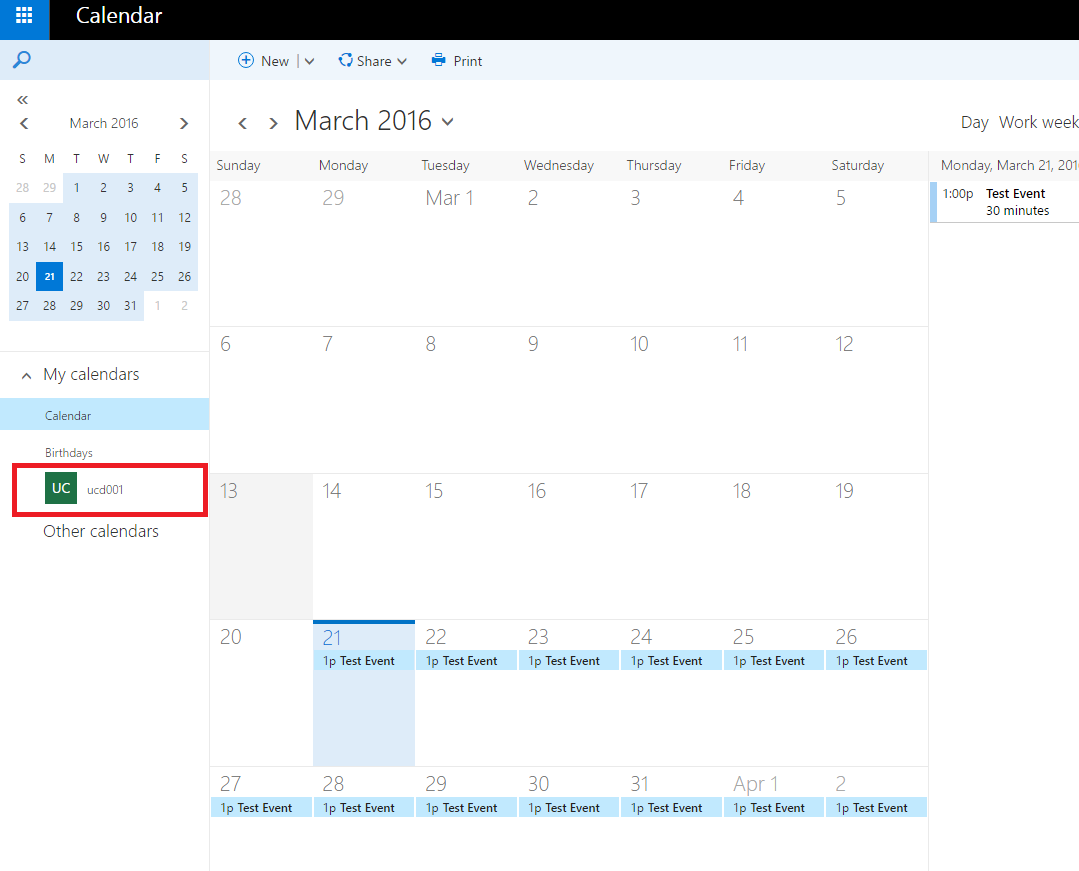The image depicts a calendar with a black banner at the top left corner featuring the word "Calendar." The month displayed is March 2016. In the calendar, a series of events are scheduled from March 21st to April 2nd, all occurring at 1 p.m. each day. These events are labeled "Test Event." The events are highlighted with a light blue line running across the top of the corresponding dates.